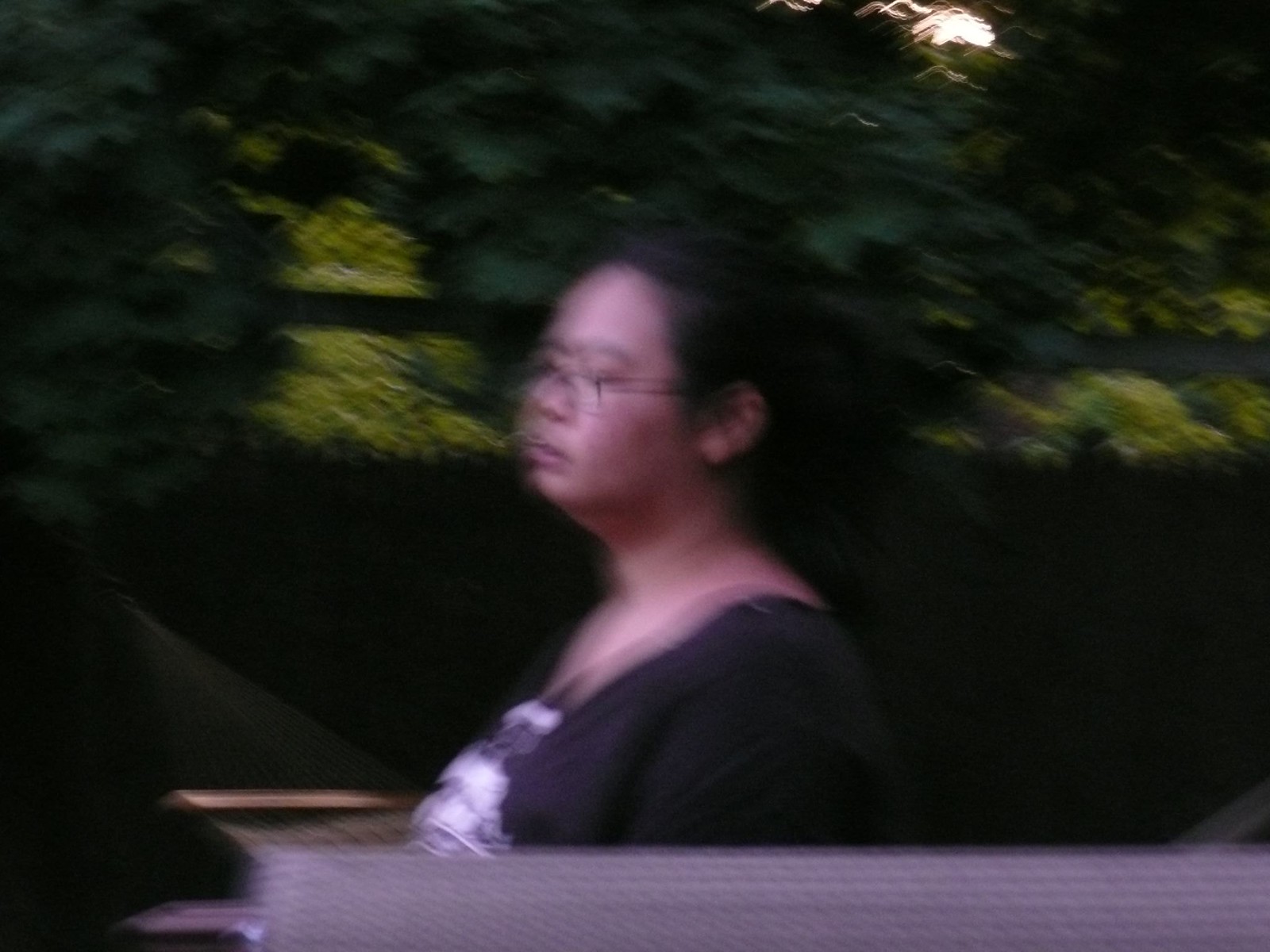In this blurry rectangular photograph presented in portrait orientation, we see a woman captured from the chest up. She is posing in a side view, facing towards the west. The woman is clothed in a black top, potentially featuring a black and white fabric detail at the center. Her gaze is directed downwards with her eyes closed, accentuated by a pair of thin, dark-rimmed glasses. Her black hair appears to be pulled back, possibly into a bun or ponytail, as it is lifted off her forehead and sides.

The background comprises muted tones of dark black, dark green, and light green, suggesting a natural setting with foliage. A strip of gray along the bottom of the photograph hints at an artificial structure, perhaps the edge of a bench she might be sitting on or a wall she is standing behind. The overall scene is softly illuminated, with light filtering through the greenery, adding a tranquil touch to the composition.